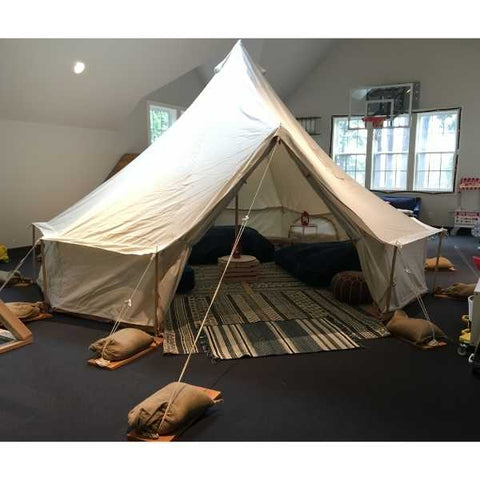In the image, a white tent is set up inside an attic-like room with angled white walls and a blue rug covering the floor. The tent, which is held down by ropes attached to brown boards weighted with various shades of brown sandbags, creates a curious indoor setup. The flap of the tent is pulled back, revealing a cozy interior with a green and white striped rug, a small black table, and possibly a black sofa and dresser. This peculiar room, featuring a three-pane window on both the left and right walls, also includes a basketball hoop with a clear backboard and an orange rim positioned above a set of three large windows. A chair can be seen against the right wall, adding to the room's eclectic mix of furnishings.